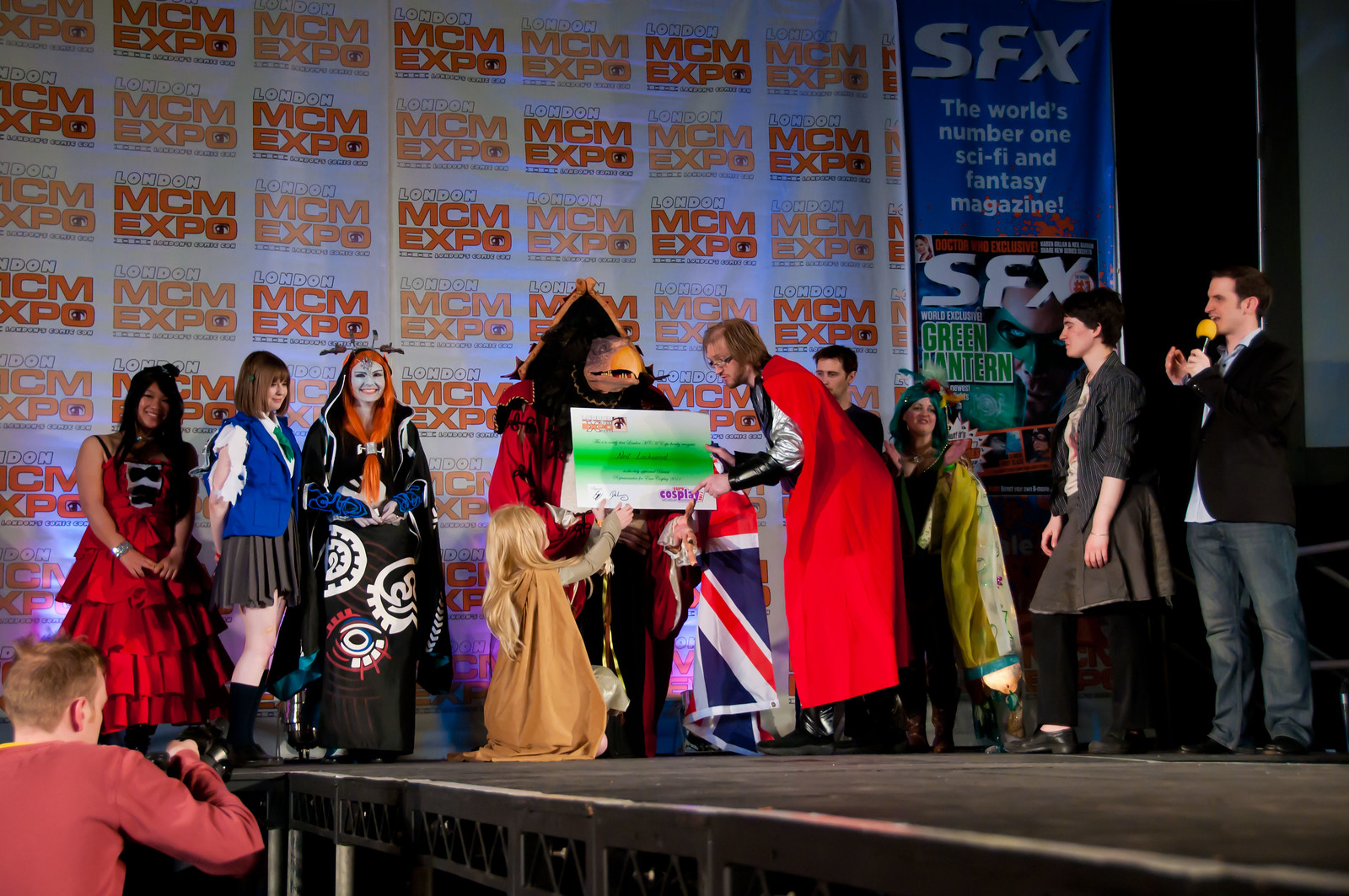The image captures a vivid and diverse group of approximately ten individuals standing on a black stage at the MCM Expo, as indicated by the repeating red and orange "London MCM Expo" sign in the background. This gathering seems to resemble a cosplay event or costume contest. From left to right, the lineup includes a woman in a frilly red dress, followed by another in a black pleated skirt and blue vest paired with a white top. Next to her stands a woman donning an orange wig and a dark cape. Central to the group is an individual wearing a dinosaur mask with a beak, clad in a black and red cloak, receiving a large certificate from a man in a silver outfit and a red cape, who has shoulder-length brown hair and black-framed glasses. Notably, a blonde woman in a brown robe kneels nearby, reaching for the certificate. Completing the scene, there's a man in contemporary attire featuring a blazer and blue jeans holding a yellow microphone, and a woman beside him with black hair, dressed in a gray shirt, skirt, and black shoes. The overall image exudes a festive, eclectic vibe indicative of the celebratory spirit of the Expo.